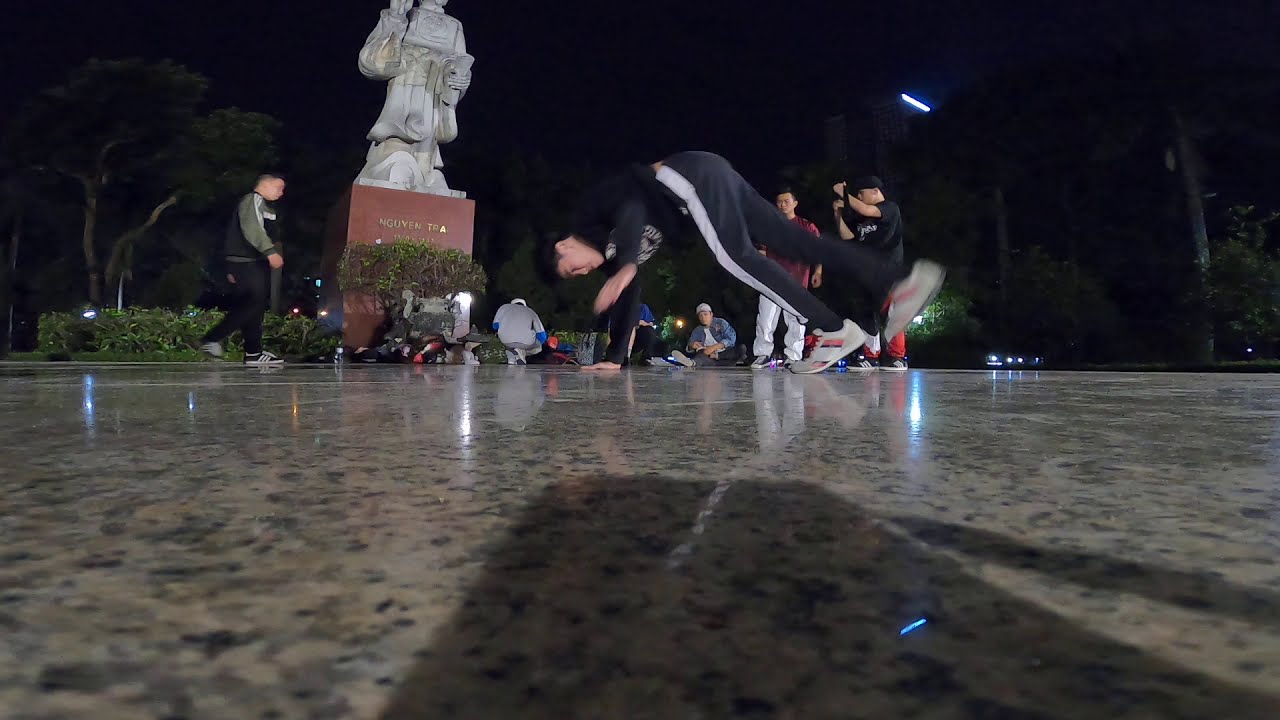In this dynamic nighttime scene set in a brightly lit courtyard with polished marble or granite flooring, a breakdancer is captured in mid-performance, pushing himself up from the ground. His right hand is firmly planted on the shiny, tan surface speckled with black, while his left hand is raised in the air. He's wearing a black jumpsuit with white stripes running down the legs. His arched body suggests he's about to execute a spin or handstand. His face is visible, turned slightly towards the viewer. In the background, a group of onlookers, some seated and others standing, can be seen observing the performance. The seated individuals are mostly dressed in gray, with one wearing a black jacket. A man in black pants and a dark green shirt is walking towards the crowd on the left. Nearby, a man in a red short-sleeve shirt and white pants stands next to another with a black shirt, black hat, and red pants, possibly capturing the performance with a camera. Also notable in the background is a prominent dark-colored statue of what appears to be a priest holding up their right arm and holding an object in their left hand, along with a few trees and lighting elements enhancing the nighttime ambiance.